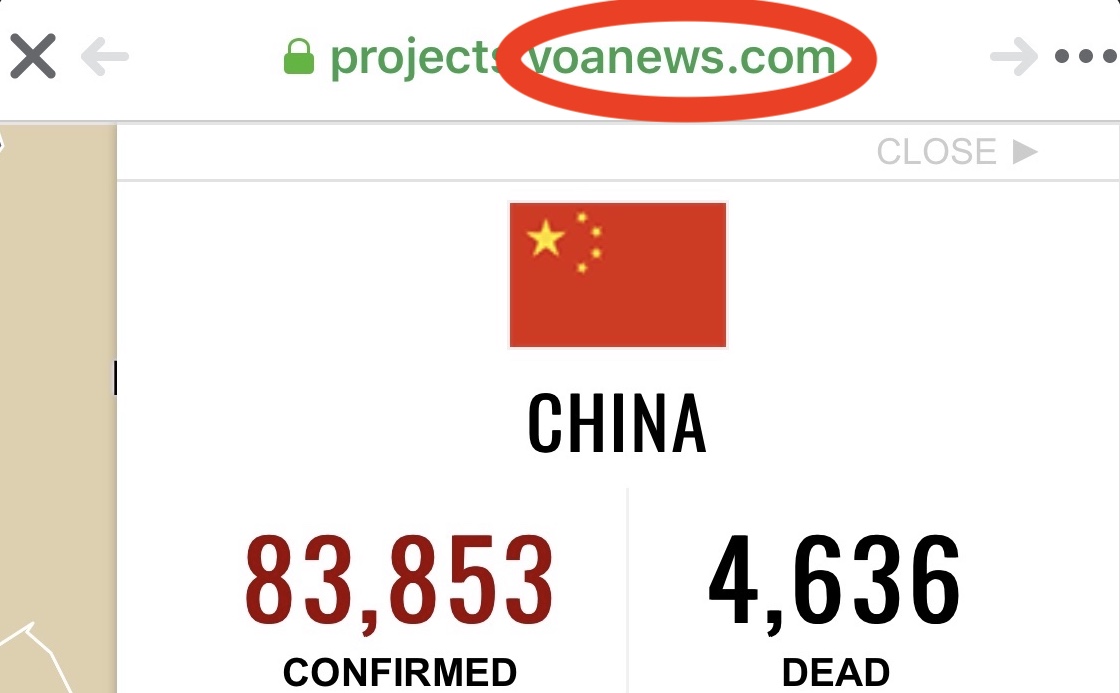A horizontal image captured from a smartphone is displayed on a white computer screen background. The interface features multiple design elements. 

In the top left corner, there is a block 'X' and a gray arrow pointing left, along with a small lock icon in the center. The URL "ProjectsVillainNews.com" is prominently displayed in green, with "Villain News" circled in red. On the right side is a gray arrow and three horizontal dots.

A thicker tan rectangle is present on the left edge of the image, while the right edge features a thin gray-black line. A gray bar runs across the top, but certain elements extend above it, leaving the topmost part clear. Below that, it reads "Close" with an arrow pointing right.

In the main content area, a red square featuring five yellow stars, representing the Chinese flag, is centered on a white background. Beneath the flag, the word "CHINA" is written in bold, black uppercase letters. 

A maroon line separates two sections of text below the flag. On the left, "83,853" is bolded and accompanied by the label "Confirmed" in black text. On the right, "4,636" is similarly bolded, with "Dead" written in small black uppercase letters underneath.

This structured and detailed description captures the design and information presented in the image.